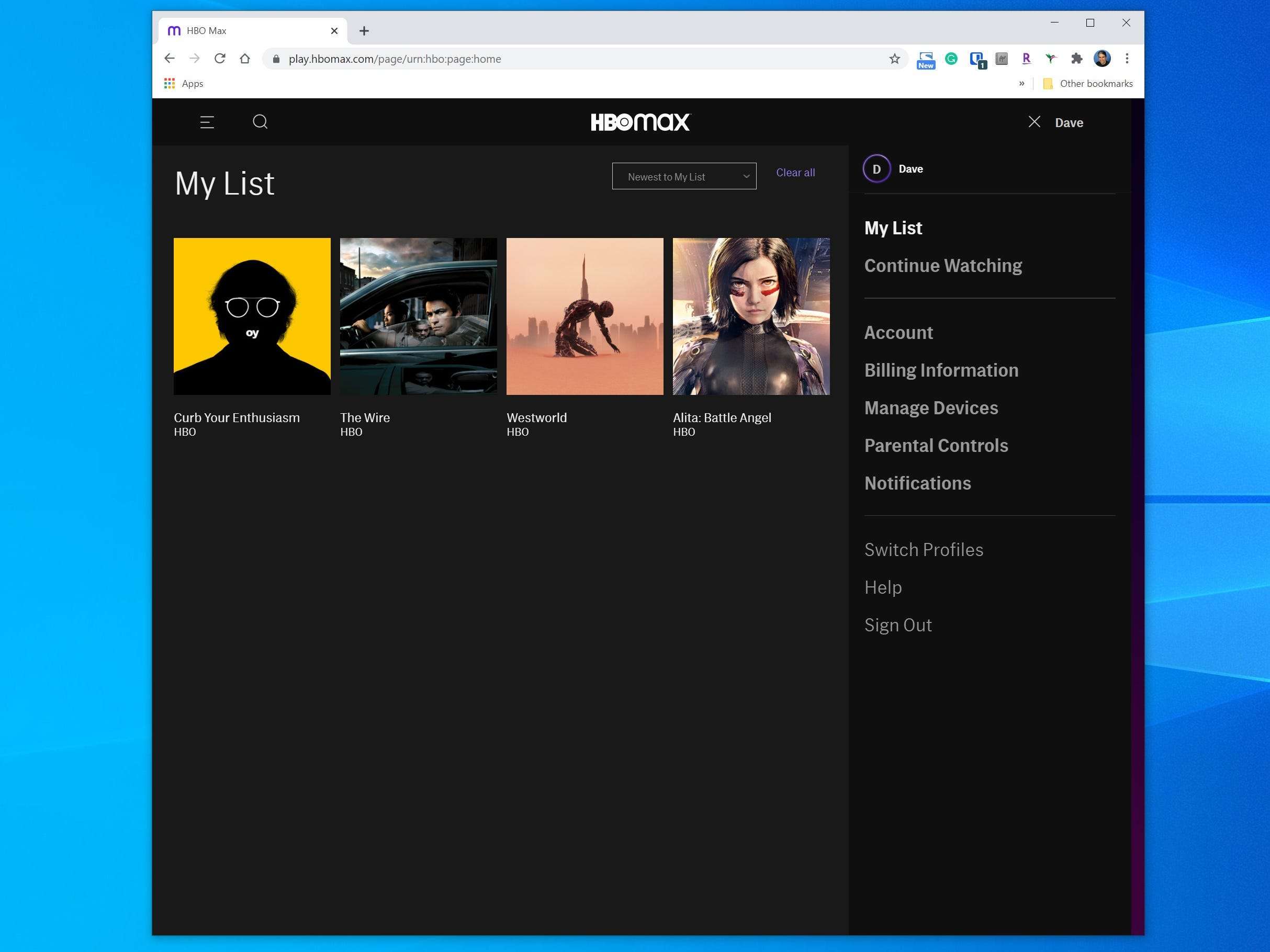The screenshot displays the HBO Max homepage on the web (play.hbomax.com/page/HBOpagehome). The top navigation bar includes several icons: a gray box with a minus sign, a square with an 'X', left and right arrows, a refresh button, a home icon, and HBO Max branding. Below the top navigation bar, there are various icons labeled sequentially from 1 to 9. 

The primary content area shows the user's customized list titled "My List," featuring popular shows and movies such as "Curb Your Enthusiasm," "The Wire," "Westworld," and "Alita: Battle Angel." The artwork for "Alita: Battle Angel" is highlighted, depicting a digital drawing of the protagonist in a skin-tight suit.

On the left sidebar, there are links for different user options, including "My List," "Continue Watching," "Account," "Billing Information," "Manage Devices," "Parental Controls," "Notifications," "Switch Profiles," "Help," and "Sign Out." 

The background of the page features a blue wallpaper design, creating a sleek and modern aesthetic for the streaming platform's interface.